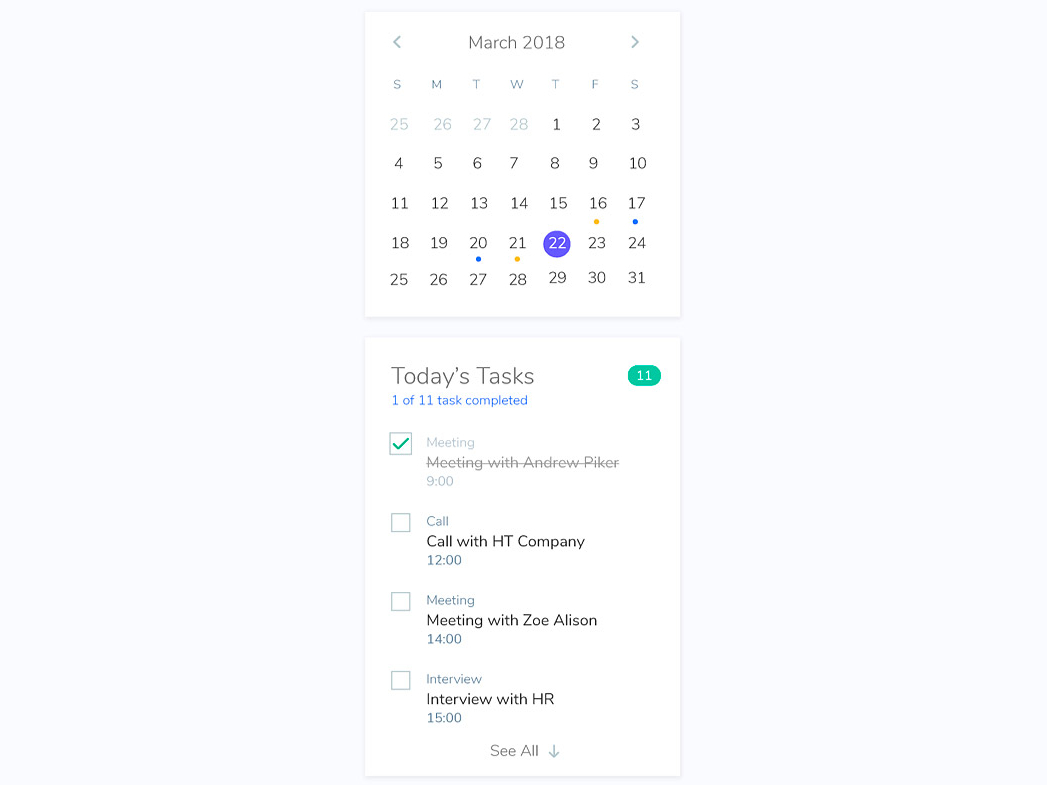**Image Description: Detailed View of Calendar Style App (March 2018)**

The image showcases a two-panel interface from a calendar-style app. The top panel features a square, white background with black text, displaying the month "March 2018" at the top. Directly below the month name is a row of headings for the days of the week abbreviated as S, M, T, W, T, F, S. The dates 25-26 and 27-28 are shown in a grayed-out font, indicating they belong to the previous and following months, respectively. The numbers from 1 to 31 are displayed in black font, representing the days of March.

Interspersed among the dates, several days have small colored dots beneath them, denoting special events or reminders:
- March 16 has an orange dot.
- March 17 has a blue dot.
- March 20 has a stark blue dot.
- March 21 has a peach-colored dot.
- March 22 features a purple circle with the number 22 superimposed on it.

The bottom panel is a vertical pane titled "Today's Tasks." On the right side of this header is a mint green oval stating the number 11, likely indicating the number of tasks for the day. Below this title, there's a statement "One of 11 tasks completed."

Four tasks are listed below with corresponding radio buttons:
1. The first task, "Meeting with Andrew Heicher, 9:00 AM," is checked off with a green check mark and the text is struck out.
2. The next task is "Call with HT Company, 12:00 PM," displayed in bold text.
3. The following task is "Meeting with Zoe Allison, 2:00 PM," also in bold.
4. The final visible task is "Interview with HR, 3:00 PM," similarly in bold.

At the very bottom of the pane, there is an option labeled "See All" with a downward-pointing arrow, indicating that more tasks are available on expanding the list.